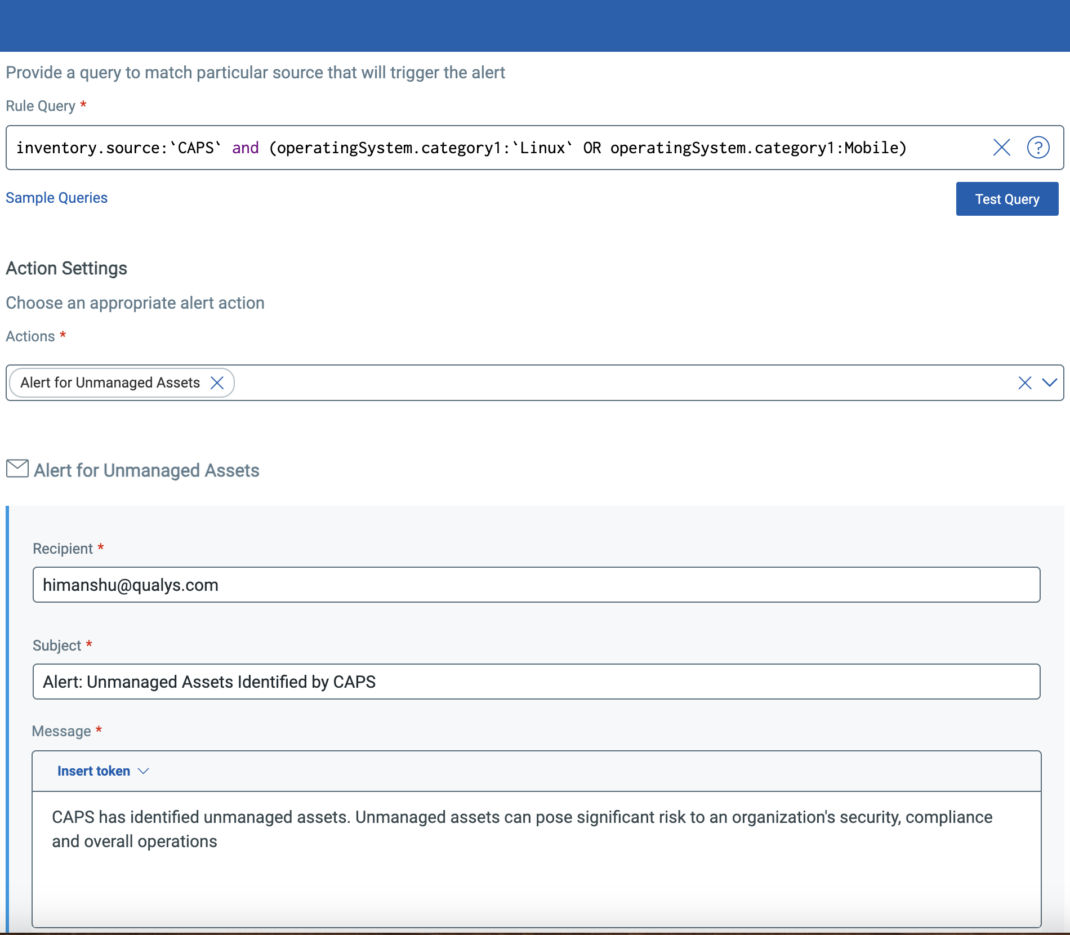This image displays a section of a web interface designed for configuring alert rules based on specific query criteria. At the top, a dark blue strip runs horizontally across the screen. Underneath, the text reads "Provide a query to match a particular source that will trigger the alert" in gray on a white background. Following this, "Rule Query" is indicated with a red asterisk marking it as a required field.

A text box below this directive contains the example query in black text: `inventory.source == 'CAPS' && (operatingSystem.category1 == 'Linux' || operatingSystem.category1 == 'mobile')`. To the right of this text box are clickable icons: a blue cross (presumably for closing or clearing the field) and a blue question mark inside a circle indicating help or information is available.

Beneath this section, the label "Sample Queries" is highlighted in blue text, suggesting it is a hyperlink. On the far right, there is a blue rectangle button with "Test Query" written in white, providing the option to test the given query.

The next section down is labeled "Action Settings" with the subtitle "Choose an appropriate alert action." Within this section, under the "Actions" header, another required field is indicated by a red asterisk. A selectable or typable box beneath it is pre-filled with "Alert for unmanaged assets." Below this field, there is an envelope icon indicating email settings.

The image also includes the option to compose and send alert messages, with an example recipient email address: himanshu@qualis.com.